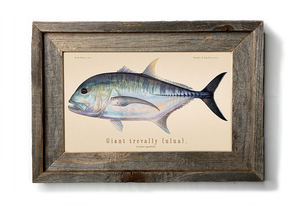This is a close-up photo of a framed art print of a fish, encased within a thick, rustic, weathered wooden frame with multiple textures. The frame, which is rectangular and shorter on the sides than on the top and bottom, casts a shadow on the white wall it's mounted on. The artwork inside features a detailed side view of a small fish against cream-colored, off-white paper. The fish is predominantly blue with a white belly and exhibits silver and green hues, along with distinctive blue striped scales. Its tail is primarily black, and it has a skinny, pointed fin on its side. The fish's blunt head is characterized by a black and yellow eye and an open mouth. The scales around its gill area show a modeled discoloration of gray and white. Two dorsal fins decorate its back, with the larger positioned further back, and a single fin is present on the bottom towards the rear. Below the fish, its name is indicated in very small letters.